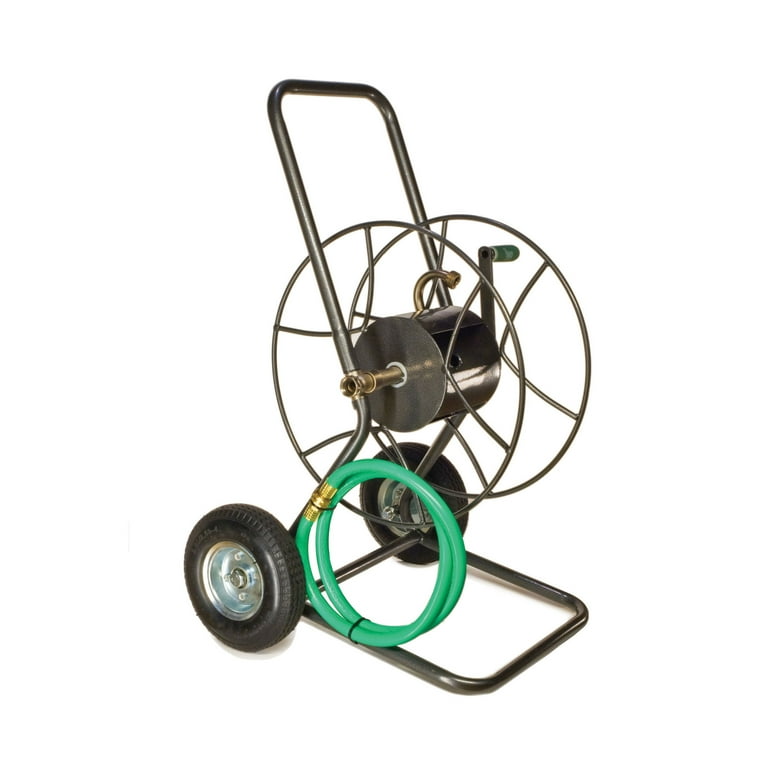The image showcases a detailed photograph of a portable garden hose organizer, also known as a hose wheel cart. This robust gardening tool features a dark green metallic frame with two rubber tires mounted on steel or aluminum rims for easy mobility. The centerpiece of the cart is a large, circular crank mechanism designed for winding the attached green hose neatly. The hose wheel cart also includes an ergonomic handle that extends from the frame, enabling the user to tip and push the cart effortlessly. The base of the cart is square with rounded edges, ensuring stability on various surfaces. The entire setup is primarily colored in shades of green and gray, and the background of the image is stark white, emphasizing the detailed design and functionality of the cart.